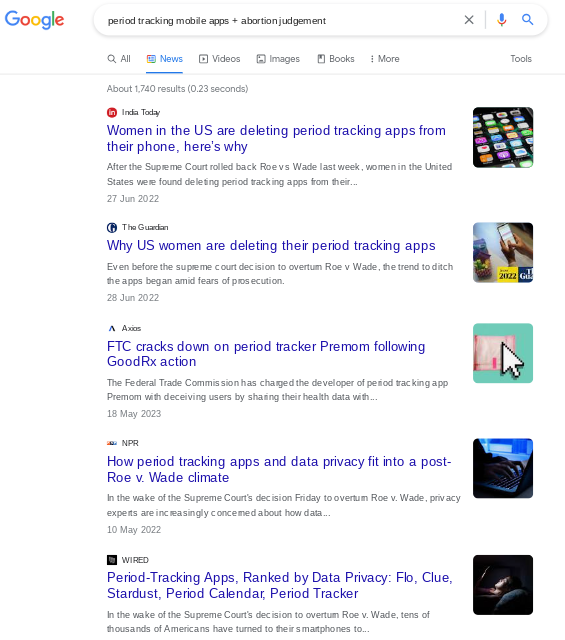The image displays a Google search results page viewed on a device with a tablet-like aspect ratio. The search query entered is "period tracking mobile apps plus abortion judgments," yielding approximately 1,740 results in 0.23 seconds. The first search result is an article from "India To Do," titled "Women in the U.S. are Deleting Period Tracking Apps from Their Phone. Here's Why." The second result is from "The Guardian," with the headline "Why U.S. Women Are Deleting Their Period Tracking Apps." The third entry is from "Axios," reporting "FCC Cracks Down on Period Tracker App Primome Following GoodRx Reaction." The fourth result from "NPR" discusses "How Period Tracking Apps and Data Privacy Fit into a Post-Roe v. Wade Climate." The final result is an article from "Wired" titled "Period Tracking Apps Ranked by Data Privacy: Flo, Clue, Stardust, Period Calendar, and Period Tracker."